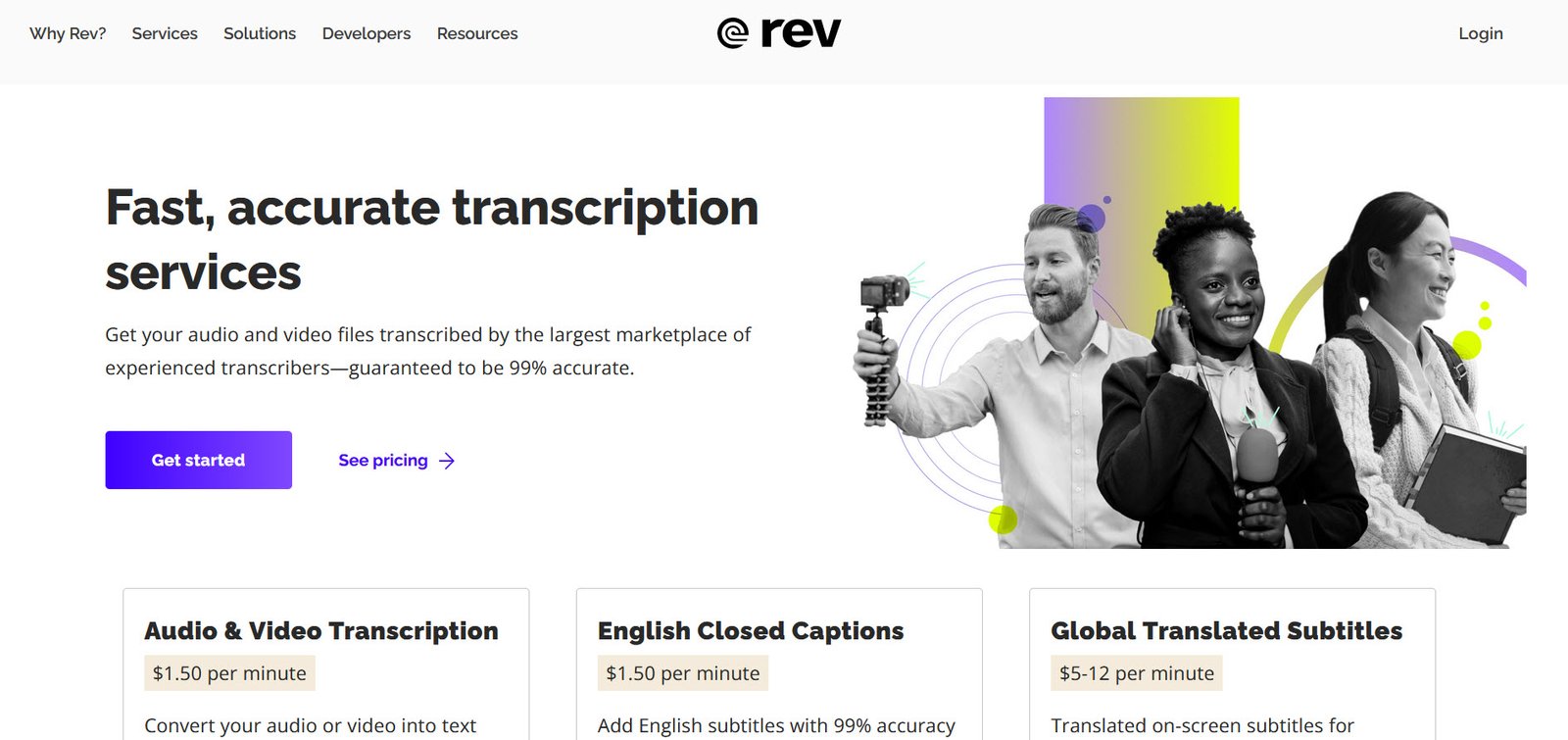The screenshot captures the homepage of Rev, a company specializing in transcription and subtitle services. Positioned to the left of the company name "Rev," all in lowercase, is a unique symbol resembling an at symbol. On the left side of the webpage, there is a navigational menu with the options: "Why Rev?", "Services," "Solutions," "Developers," and "Resources." To the right, there's a login button.

The central part of the screenshot features a vibrant stock photo illustrating a diverse group of people. A white male, holding a camera on a selfie stick, appears to be filming himself. To his left, an African-American woman with dreadlocks is smiling while holding a microphone and adjusting an earpiece. To her left stands an Asian woman, also smiling, with a heavy, hard-bound book in one hand and a backpack slung over her shoulder.

Beneath the photo, the text promotes Rev’s core services: "Fast, accurate transcription services. Get your audio and video files transcribed by the largest marketplace of experienced transcribers, guaranteed to be 99% accurate." Below this statement, a prominent purple button invites users to "Get Started," and alongside it, purple text with an arrow encourages them to "See Pricing."

Further down, three pricing options are listed for the services offered:
1. Audio and Video Transcription at $1.50 per minute – Convert your audio or video into text.
2. English Closed Captions at $1.50 per minute – Add English subtitles with 99% accuracy.
3. Global Translated Subtitles at $5-12 per minute – Translated on-screen subtitles (with more detailed pricing cut off).

The screenshot ends here, without additional content below these services.